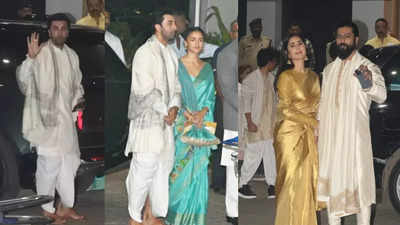This image collage features three side-by-side photographs capturing the vibrant essence of an Indian wedding celebration. 

In the left photograph, we see a man standing in front of a sleek black SUV, dressed in traditional white attire consisting of loose pants and a tunic. He sports black hair, a beard, and a mustache, and is waving cheerfully at the photographer.

The center photograph showcases a couple standing together. The woman is elegantly attired in a bright turquoise blue sari with a shimmering gold edging, featuring a V-neck design. Her black hair is impeccably styled into a bun. Standing next to her is the same gentleman from the first photo. He is now adorned with a white shawl accented by silver tassels draped around his shoulders.

On the right, another couple is pictured. The woman dazzles in a metallic gold sari with an even brighter gold border, complementing her long, flowing dark hair and gold dangle earrings. Beside her stands a man with an impressive long black beard and mustache, dressed similarly in a white tunic over white pants with a matching white shawl around his neck. He, too, waves warmly at the camera.

Together, these images beautifully capture the joyous and colorful spirit of an Indian wedding celebration.